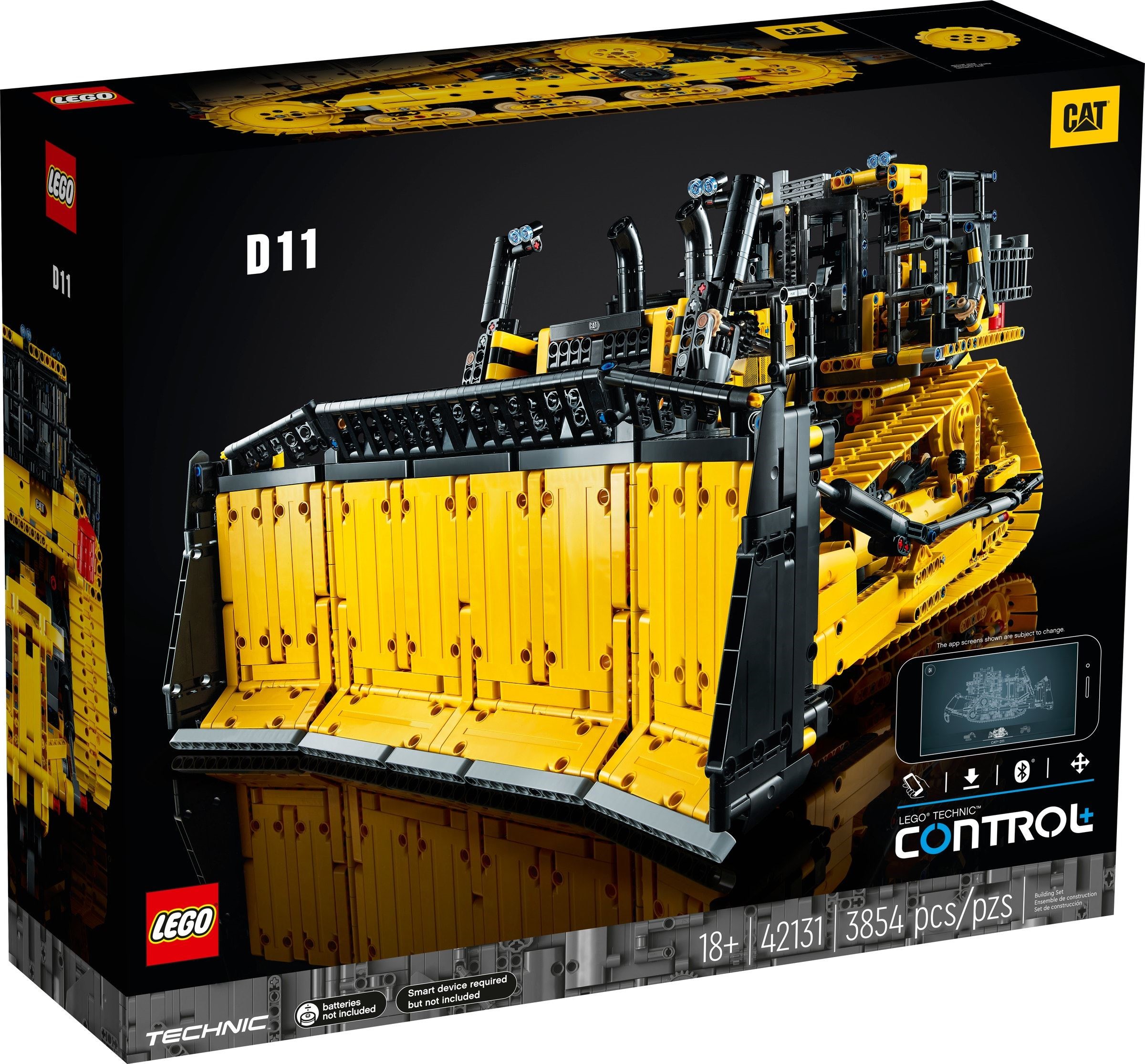The image depicts the packaging of an intricate Lego Technic set designed to build a detailed replica of a Cat D11 bulldozer. The box is predominantly black and yellow, consistent with the construction theme. On the top right corner, there is the recognizable Cat logo, and on the upper left, it reads "D11". The bottom left corner features the iconic red Lego logo with white font. The bulldozer model showcased on the front of the box is largely yellow with black accents, featuring a large flat scoop at the front used for bulldozing dirt, and detailed components like pipes and exhausts built from specialty Lego parts. The machinery, outfitted with yellow tank treads around its wheels, has a cabin space for an operator. Notably, this set contains 3,854 pieces, as indicated on the bottom of the box. The lower right specifies compatibility with the Lego Technic Control Plus app, suggesting that the setup includes a smartphone interface to assist in building and operating the model. Additional specifications include "batteries not included," "smart device required but not included," and an age recommendation of 18 years or older. Overall, the packaging reflects a highly articulate and elaborate Lego set aimed at advanced builders.